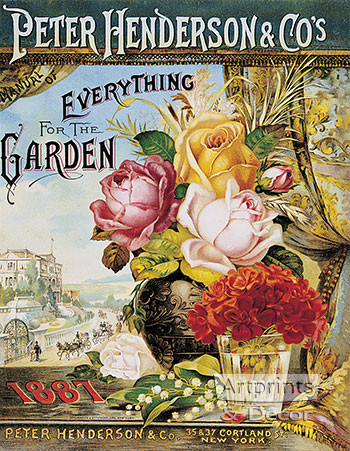This art print from 1887 features a vibrant bouquet of flowers set against a light blue background. At the top, in an old-fashioned black font, it states, "Peter Henderson and Company," with a subheading, "Everything for the Garden." The central focus is a combination of a large brown vase and a basket, both brimming with flowers. In the arrangement, you can find red, pink, yellow, and off-white roses dominating the display. Additionally, another vase contains orange-red flowers. The print has a somewhat faded, vintage look, enhancing its historic charm. There's a hint of intricate detail in the background, where a building and horse-drawn carriages are faintly visible, giving the impression that the flowers are inside while you're looking out at the scene outside. In the corner, the year "1887" is subtly marked, and at the bottom left, it reads "Art Prints and Decor." The entire composition appears to be delicately crafted, possibly using pencil and watercolor techniques, making it a visually appealing and nostalgic piece.